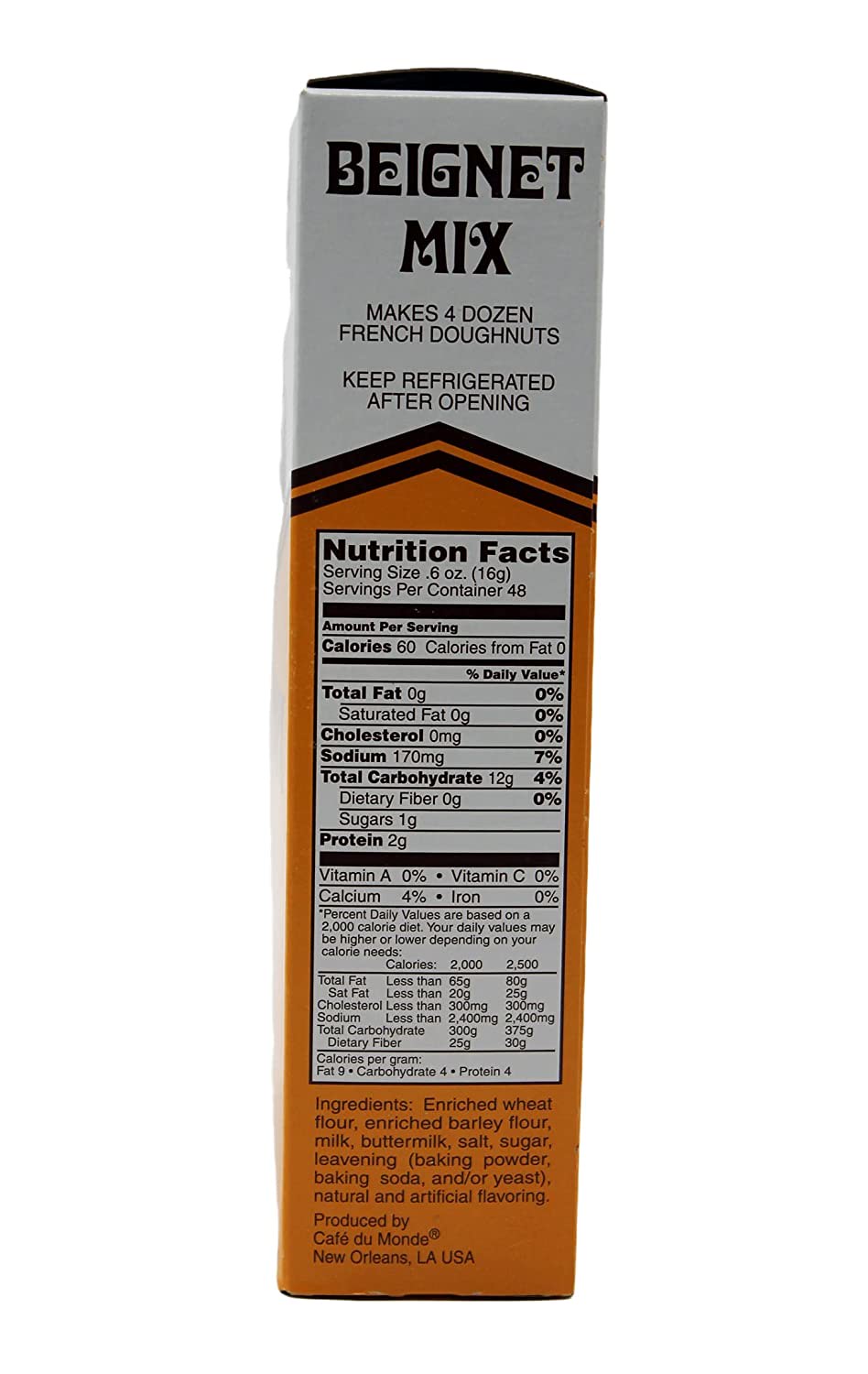This high-quality image showcases the side of a long box container for Café Du Monde Beignet Mix, prominently featuring its white and orange color scheme. The top section of the box is white, displaying bold text that reads "Beignet Mix" in a signature font, followed by "Makes Four Dozen French Donuts" and "Keep Refrigerated After Opening." Below this, the box transitions into an orange section that contains a detailed table of nutrition facts. The nutrition label specifies a serving size of 0.6 ounces, with 48 servings per container. It lists calories, total fat, cholesterol, sodium, carbohydrates, fiber, sugar, protein, vitamins, calcium, and iron. Further down is an ingredients list that includes enriched wheat flour, enriched barley flour, milk, buttermilk, salt, sugar, leavening agents (baking powder, baking soda, and/or yeast), and natural and artificial flavorings. The bottom of the box notes that the product is produced by Café Du Monde in New Orleans, Louisiana, USA. The entire image appears against an edited plain white background, giving it the appearance of an advertisement for the product.